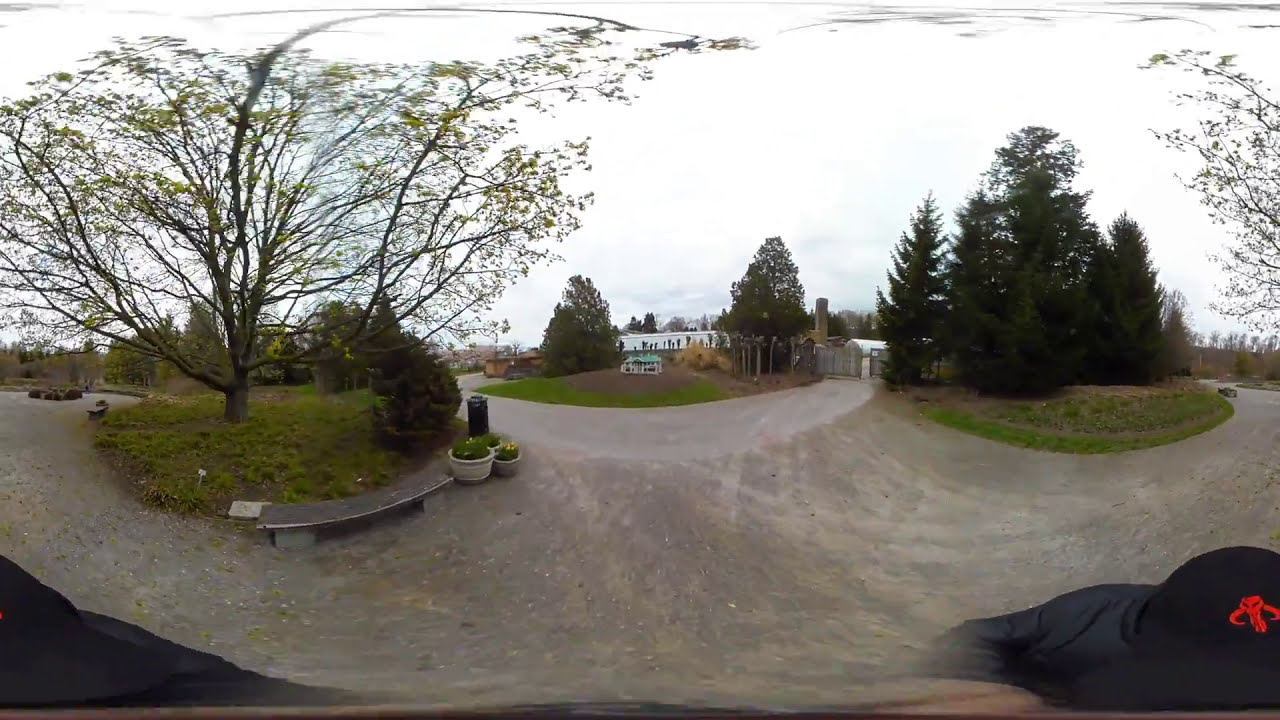The photograph is a high-quality, panoramic 360-degree outdoor view featuring a curved, gray street or driveway. The surface, either gravel or asphalt, extends in both directions, flanked by circular islands of grass. The island on the left hosts a mostly bare tree with a shrub in front and a concrete bench decked with several potted plants. The island on the right contains several evergreen trees.

In the center background, a large patch of grass leads to an ambiguous multi-storied building obscured by a couple of large evergreens; a chimney is visible projecting from the right-hand side of the building. A white structure, possibly a gazebo or shed, stands closer in the foreground. 

The sky is overcast, lending a gray tone to the scene, though the setting remains brightly lit by natural light. The bottom right corner captures part of the photographer, donning a blue cap adorned with a red devil logo, and a dark jacket. The overall image combines elements of nature and architecture in a clear, detailed snapshot of an outdoor space.